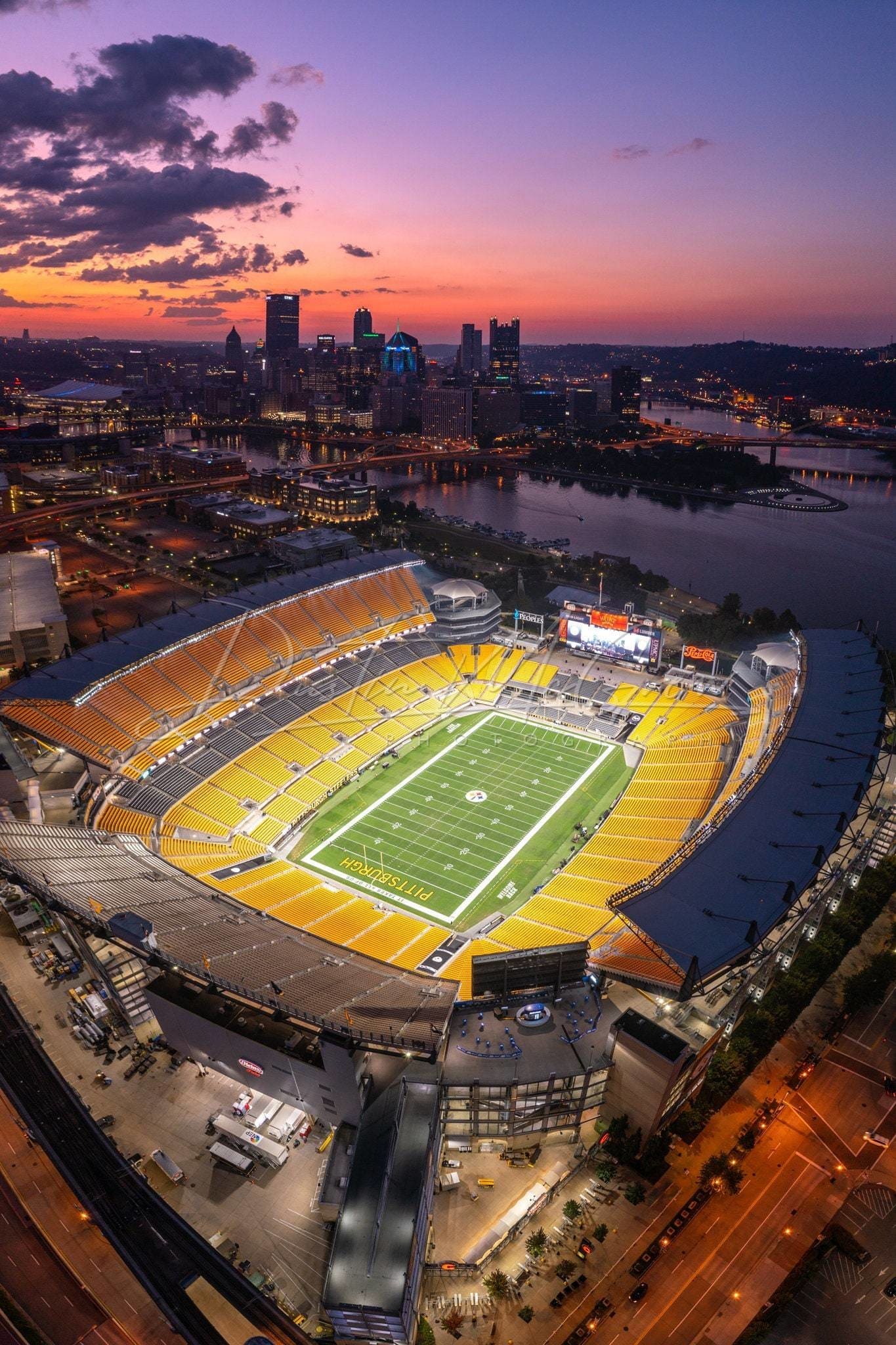This captivating aerial shot captures a lit-up football stadium in Pittsburgh, showcasing its vibrant green grass field with "Pittsburgh" inscribed on it. The seating around the stadium is predominantly yellow and white, arranged in a coliseum style. Beyond the stadium, the bustling cityscape of Pittsburgh is visible alongside meandering rivers and major freeways. The atmosphere is enhanced by a stunning sunset, painting the sky in hues of orange, purple, and red, accompanied by dark clouds. The stadium, likely belonging to either the Pittsburgh Steelers or the University of Pittsburgh, is empty and brilliantly illuminated, suggesting it's either after a game or practice. The lively nightlife of Pittsburgh begins to emerge, with streetlights and car movements adding to the dynamic cityscape. The image prominently features the central field, large scoreboard, and the unique blend of urban and natural surroundings.